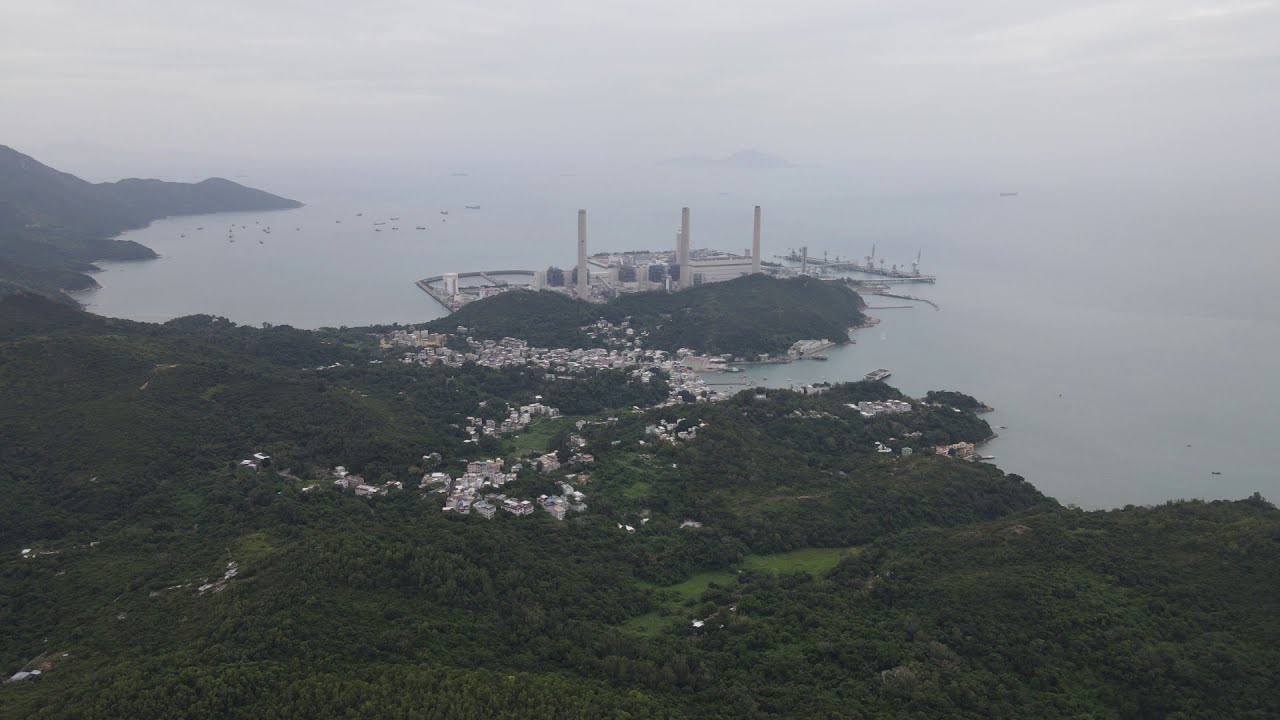The image presents a misty, overcast scene dominated by light gray skies with a few clouds, creating a hazy, potentially foggy backdrop. It appears to depict a large body of water, possibly a lake or a harbor, with water that shimmers in a silvery or gray tone, reflecting the overcast sky. In the foreground and stretching across part of the image is a forested area with many tall green trees, interspersed with several white houses and structures scattered densely throughout.

Towards the center of the picture, a green island or peninsula juts out into the water, marking a significant focal point. This island-like feature supports a large white building, which might serve as a docking area, indicated by the presence of areas that seem designed for boats to dock. Alongside this building, there appear to be several vertical poles or smokestacks, likely part of a large factory complex in the background, just behind the green protrusion.

Adding to the complexity, rocky cliffs can be seen emerging from the upper left corner, descending into the scene. This multifaceted landscape melds lush vegetation, watery expanses, and architecturally varied structures, creating a rich tapestry of natural and man-made elements.